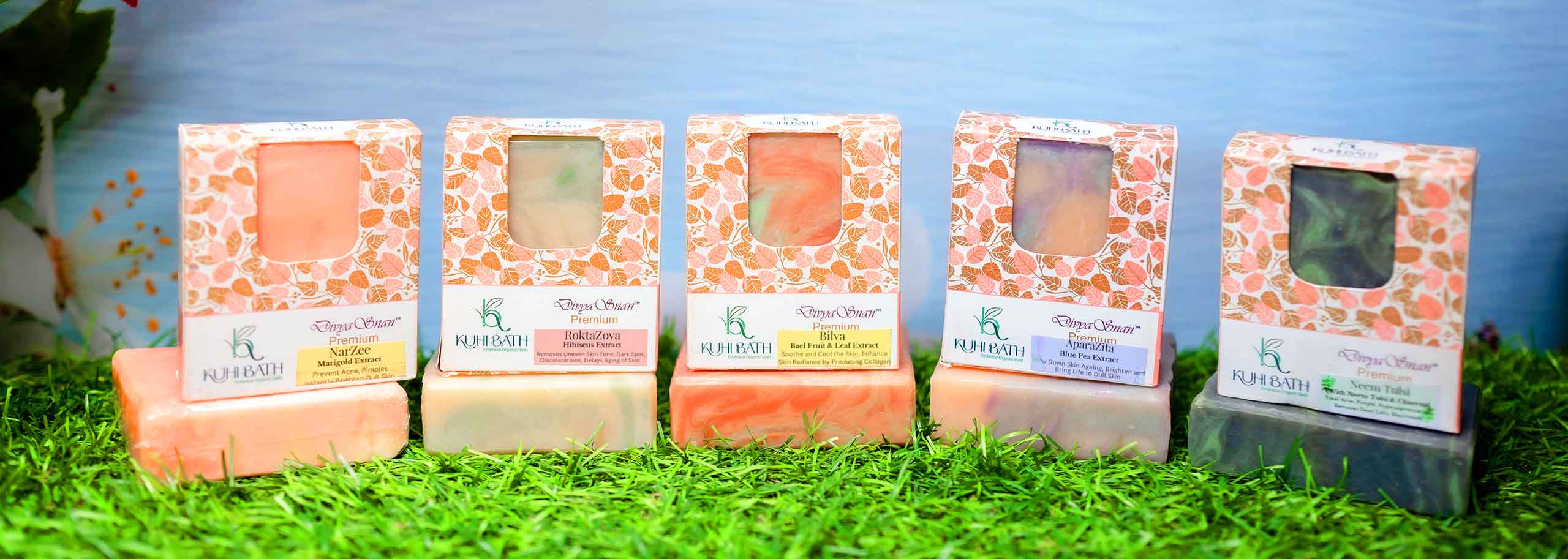This professionally-lit advertisement image showcases a collection of luxury artisan soaps displayed on faux green grass akin to Easter basket filling, set against a vibrant blue background. The soaps, presented in an elegant, semi-circular arrangement, highlight their marbled artistry with colors ranging from peach and green to blue and purple. Each bar is housed in a floral, pastel-hued box with a label, mirroring the soap's color palette. From left to right, the soaps are: a peach bar, a peach-green mix, a green with deeper peach tones, a purple-peach swirl, and a striking blue-green soap. The meticulous presentation underscores the handcrafted, bespoke nature of the soaps, evoking a sense of refined indulgence.